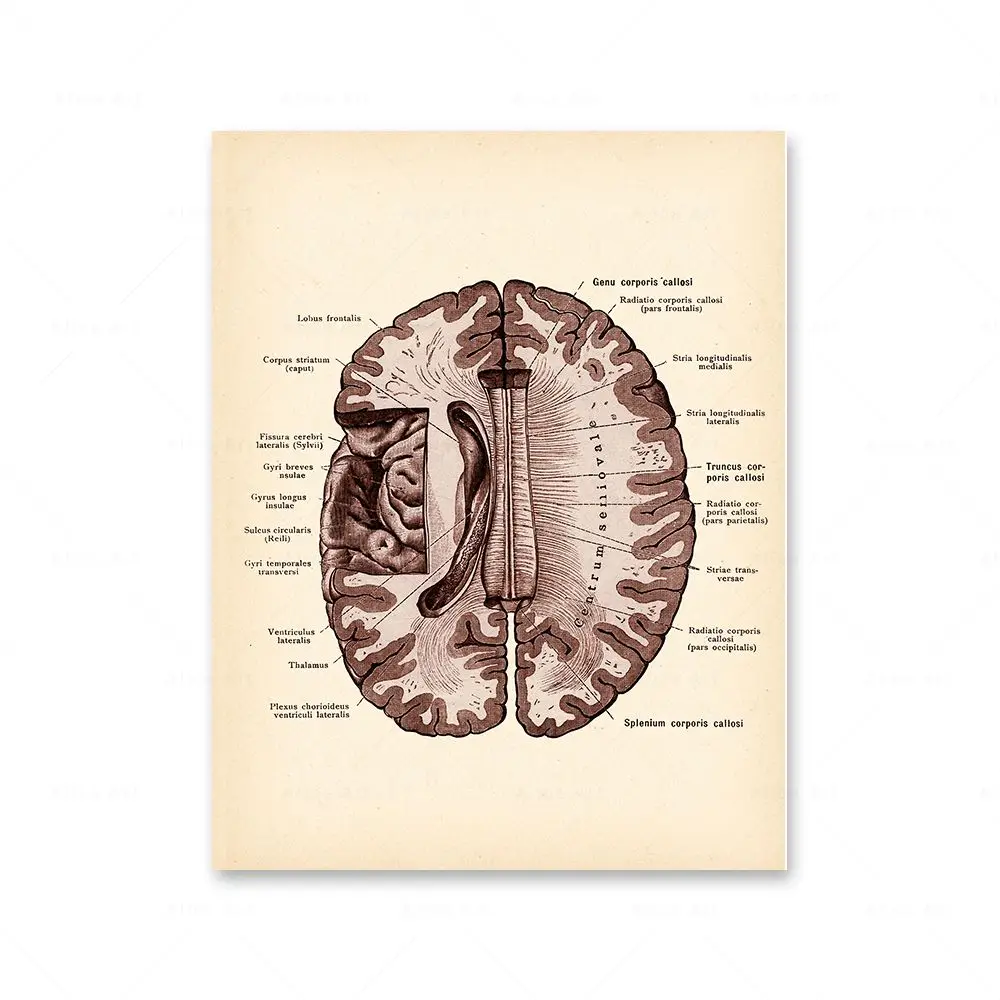The image is a cross-section of the brain, reminiscent of illustrations found in old medical books. It features a detailed portrait-style layout with the brain taking up the majority of the page, depicted in nearly grey scale with dark pink outer edges and lighter pink on the inside. The paper is an off-white, cream color, giving it an aged, yellowed appearance. The diagram extensively labels various brain segments in Latin, including terms like lobus frontalis, corpus striatum, thalamus, and splenium, using arrows to indicate specific regions. On the left side, nine sections are identified, while the right side has ten labeled areas. Prominently, the term "centrum cerebelli" is annotated within the interior of the brain, signifying a detailed examination of the brain's anatomy.